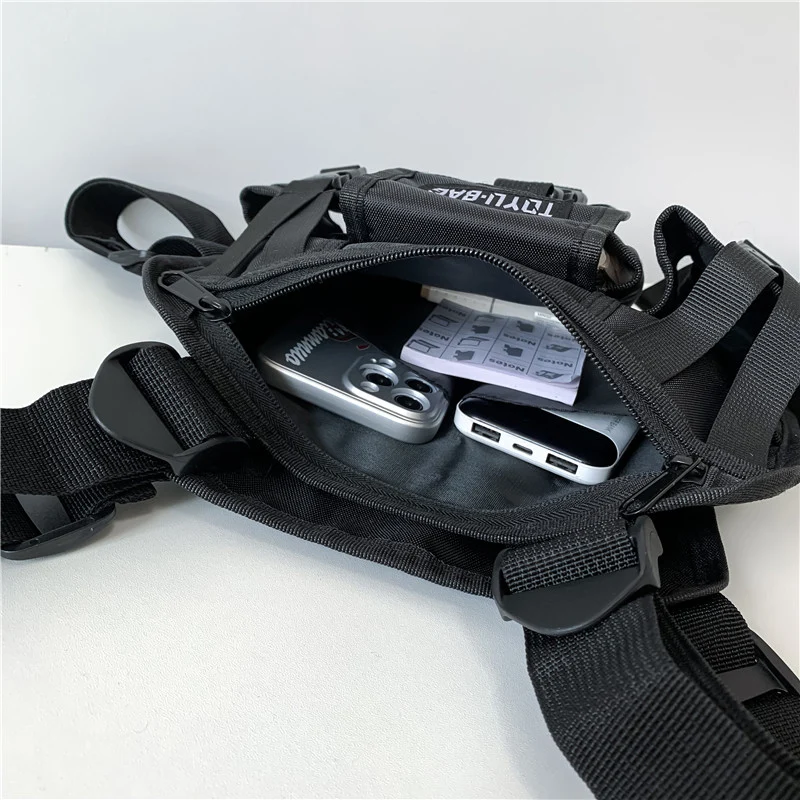The image showcases a black bag with thick, robust straps and a zipper. The bag is currently unzipped and open, revealing its contents which include two electronic devices and a small piece of paper or booklet. The bag prominently features a front pocket, which bears the name "Toyo-bag" in slightly obscure white text. Although the details of the item inside the pocket are not fully visible, there is a glimpse from the side that hints at a silver object nestled within. The overall composition of the image provides a clear and in-depth look at the bag and its contents, capturing the essence of preparedness and organization.